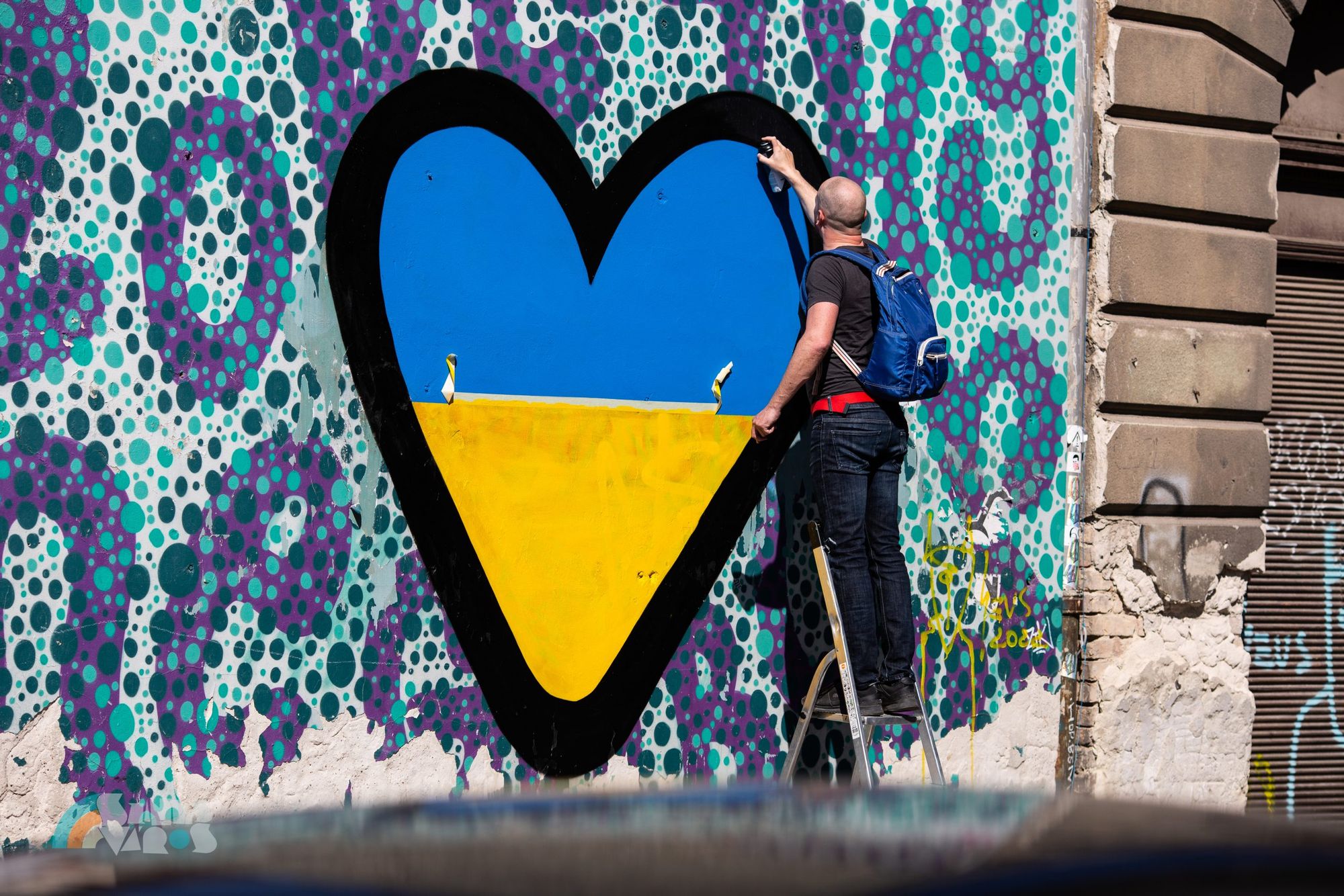The image captures a man standing on the top rung of a metal ladder, spray-painting a mural on an old city building. He wears a black shirt, dark jeans with a red belt, and a light blue backpack. His hand holds a spray can, meticulously outlining a heart that is half blue on top and half yellow on the bottom, with some masking tape slightly lifted to create a distinct horizontal separation. The heart is edged in black, adding definition. The background of the mural is a vibrant array of bubbles in various shades of blue, punctuated by purple letters, including H, Y, O, and E, adorned with dark green and teal polka dots. To the right, the building's crumbling alabaster or stone façade is visible, alongside a metal grate covered in different-colored graffiti. The man’s light skin and thinning hair are noticeable, as he focuses on completing his artwork.